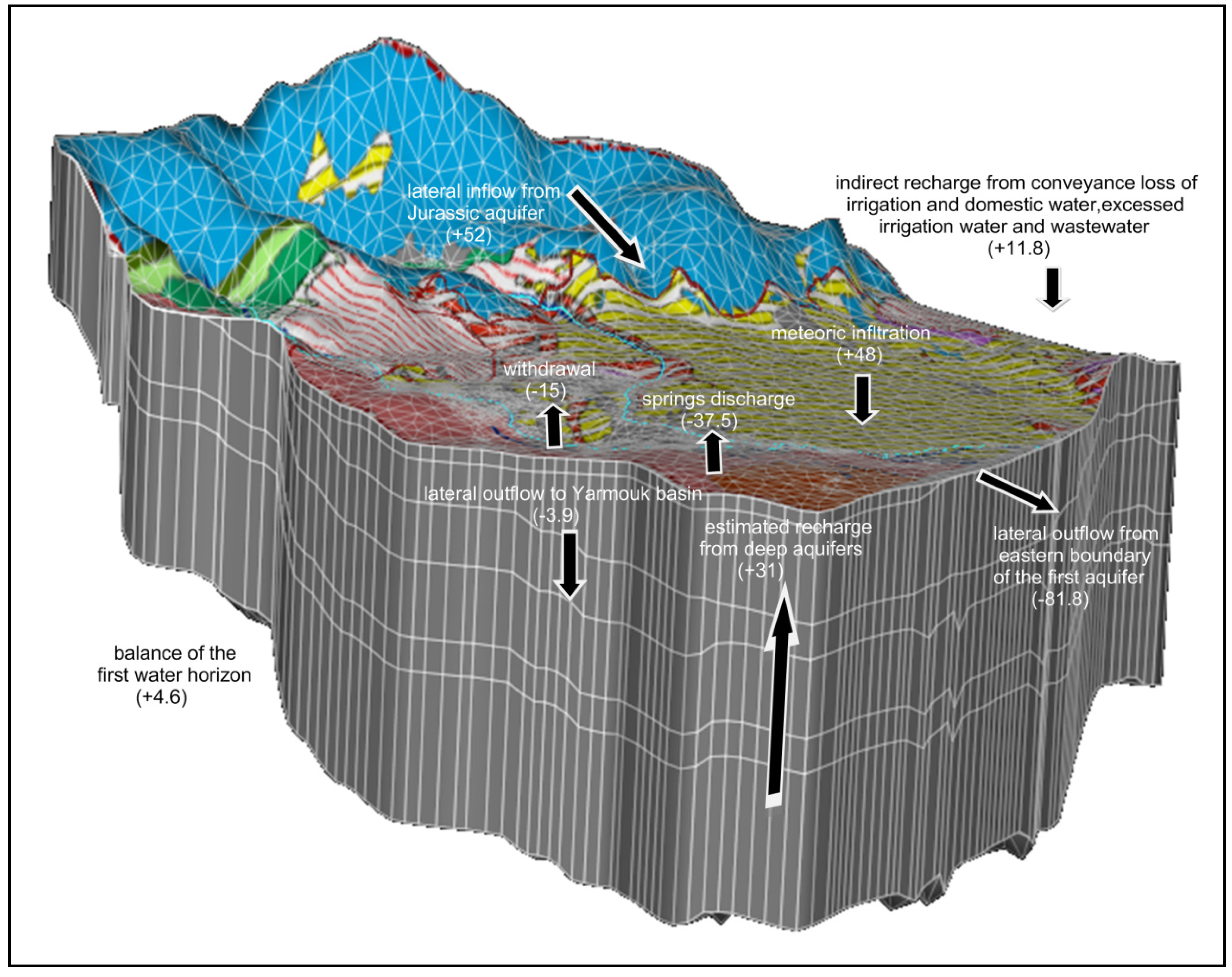This image is a detailed scientific diagram, likely of a geological structure such as a basin, showcasing both the depth and elevation of the landscape. The image prominently features various lines which provide detailed information about different heights and depths, corresponding to specific numerical values indicating elevation changes. The diagram also incorporates arrows and labels pointing to various aspects of the water cycle, including indirect recharge from conveyance loss of irrigation and domestic water, excess irrigation water, and wastewater. Additionally, there are indications of lateral inflow from a Jurassic aquifer and lateral outflow to the Yarmouk Basin, as well as estimated recharge from deep aquifers. The 3D rendering emphasizes different layers of the earth, marked by horizontal lines and shaded in various colors—blue for mountainous regions, transitioning through green, red, and finally yellow—each representing different geographic or hydrological events. This cutaway view illustrates water collection and movement within the landscape in a highly scientific and geographic context.